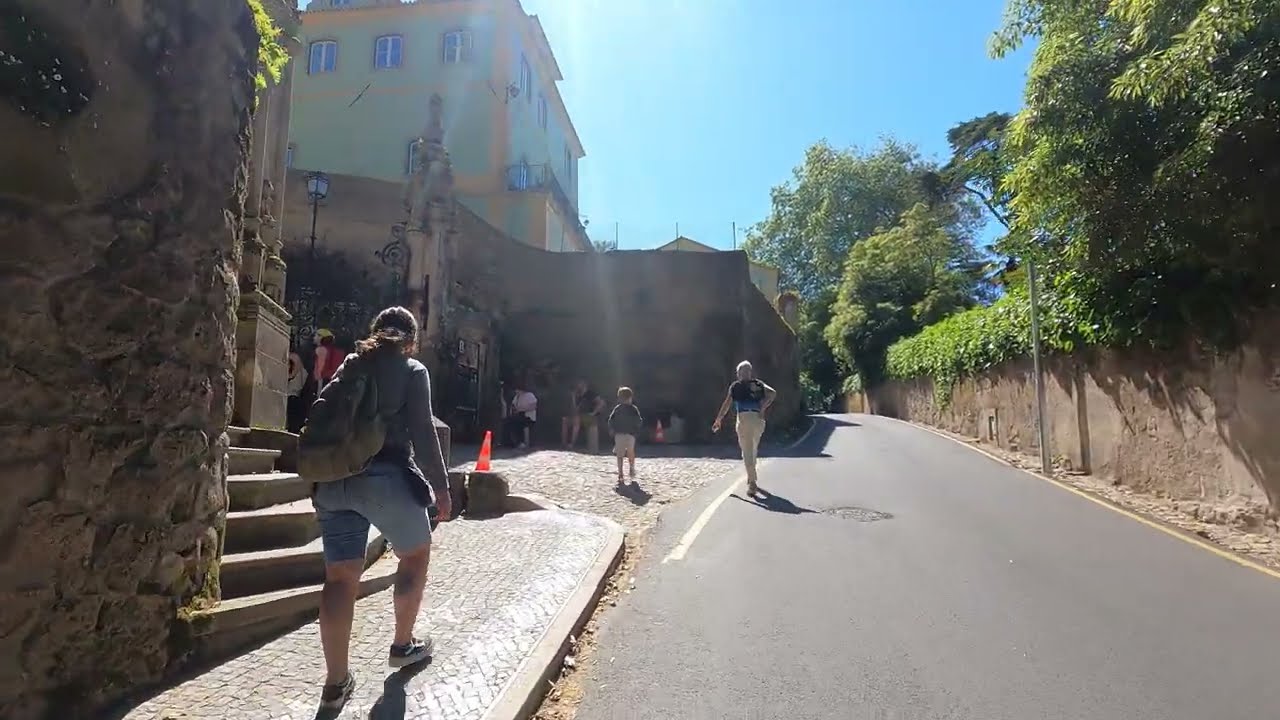This image depicts a one-lane paved street or walkway with a steep incline. On the right side, there is a tan concrete wall, approximately eight feet tall, adorned with ivy and other plants growing over and down the wall. Tall trees emerge from the top of the wall, contributing to a lush, green environment. On the left side of the photo, several buildings and a staircase are visible. People are scattered throughout, with some walking up the hill and others sitting down, likely in an outdoor restaurant area. A younger woman in jean shorts, carrying a backpack, is seen walking by herself, while an older lady and a young boy, around five years old, are also making their way up the slope. These figures are positioned near the center of the image, emphasizing their struggle with the incline. The sky is visible at the top of the image, suggesting that it is a clear day, with the photograph capturing the scene in the middle of the day. The color palette includes shades of gray, white, brown, green, blue, tan, orange, and red. Overall, the setting is an outdoor urban environment bustling with activity.